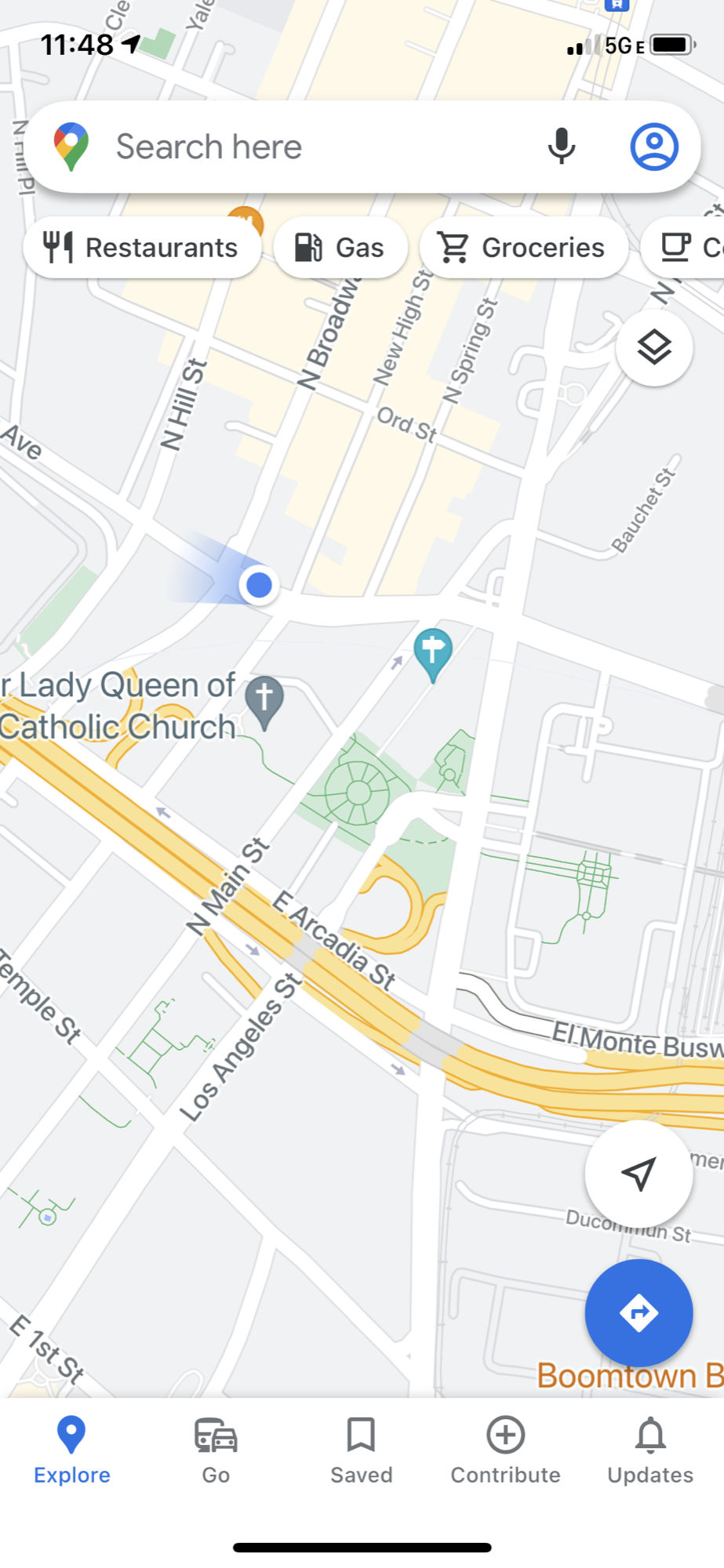A person is navigating Google Maps on their smartphone at 11:48 AM. The phone's status bar shows moderate reception with two out of four bars filled and a 5G icon. On the screen, the battery icon is black, and a white oval encompasses the Google Maps pin icon, followed by the text "Search here" in gray next to a gray microphone icon.

Further down, there's a blue silhouette icon, followed by horizontally arranged white oval tabs with black text. These tabs provide quick access to different categories: "Restaurants" marked by a fork and knife, "Gas" with a gas pump icon, and "Groceries" with a shopping cart icon. Another tab features a teacup on a saucer, partially displaying the letter "C", suggesting it may be coffee-related but is cut off due to zooming.

At the bottom of the screen, a navigation bar has the blue word "Explore," and in gray, options for "Go" with train and bus icons, "Saved," and "Contribute" with an outline of a gray circle and a white plus sign inside. A gray bell icon signifies "Updates."

On the lower right-hand corner of the map, there are two circles. The bottom circle is blue with a white diamond inside and a blue arrow pointing to the right. The top circle is white with a black arrow pointing to the upper right.

Visible street names include Los Angeles Street, North Main Street, and East Cardia Street.